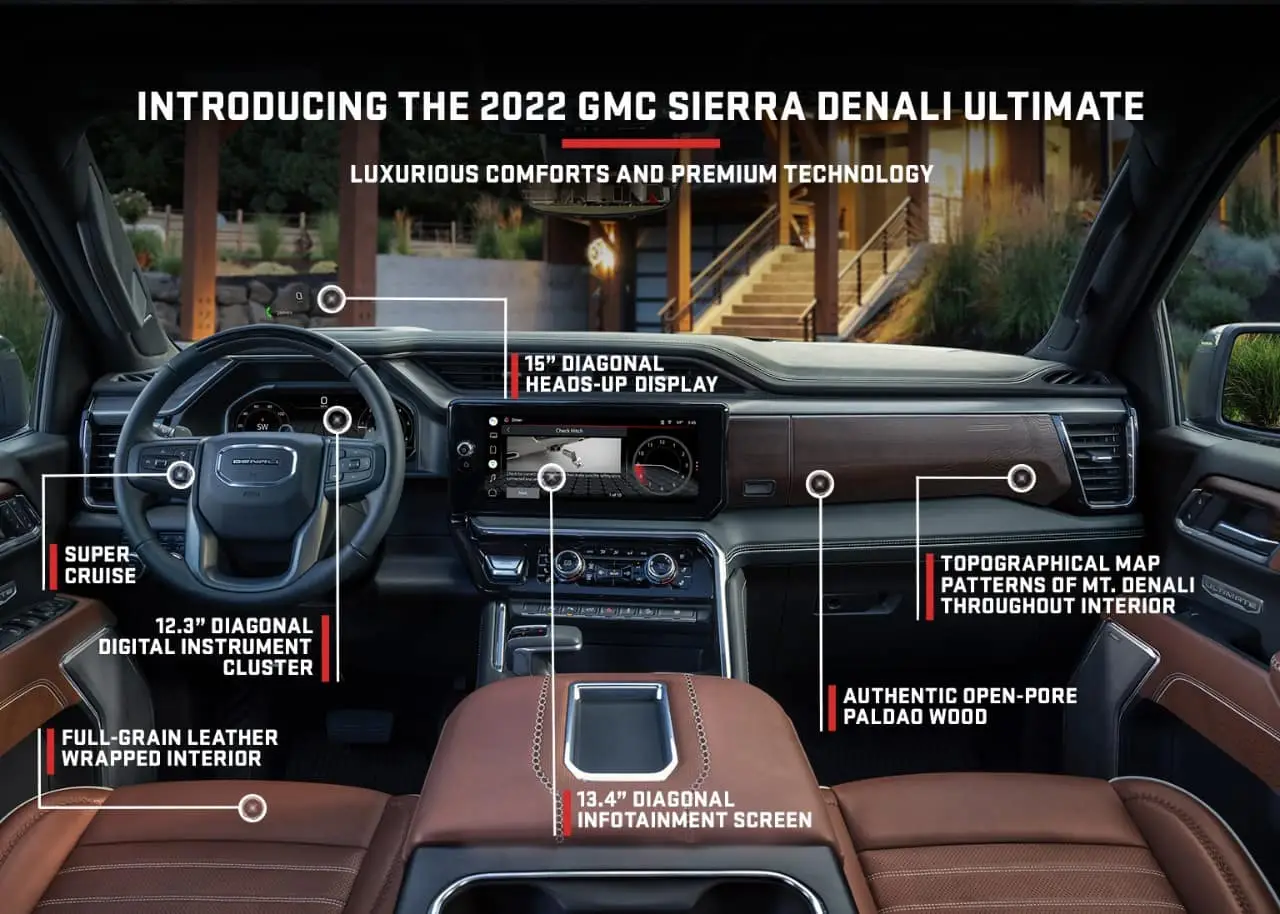Introducing the 2022 GMC Sierra Denali Ultimate, this detailed promotional image highlights the luxurious comforts and premium technology of the SUV's interior. The image showcases several advanced features with labeled lines pointing to each one. 

At the top, in bold text, it announces the vehicle model and its luxurious offerings. Starting with the left of the image, the steering wheel features Super Cruise, a hands-free driver-assistance technology. Above the wheel, you see the 12.3-inch diagonal digital instrument cluster displaying vital driving information. Behind the wheel, there is a prominent 15-inch diagonal heads-up display that projects key data onto the windshield for easy viewing.

The center of the dashboard houses a 13.4-inch diagonal infotainment system, positioned above the full-grain leather-wrapped seats that emphasize the vehicle's opulence. Authentic open-pore pale dowel wood trim adorns the dashboard, contributing to the elegant aesthetic. 

Additionally, the interior design includes topographical map patterns of Mount Denali, adding a unique and personalized touch. The vehicle's interior is visually complemented by a glimpse of the outside scenery through the windows, where you can see a house with lights and surrounding greenery, emphasizing the sense of tranquility and luxury wherever the vehicle is parked.